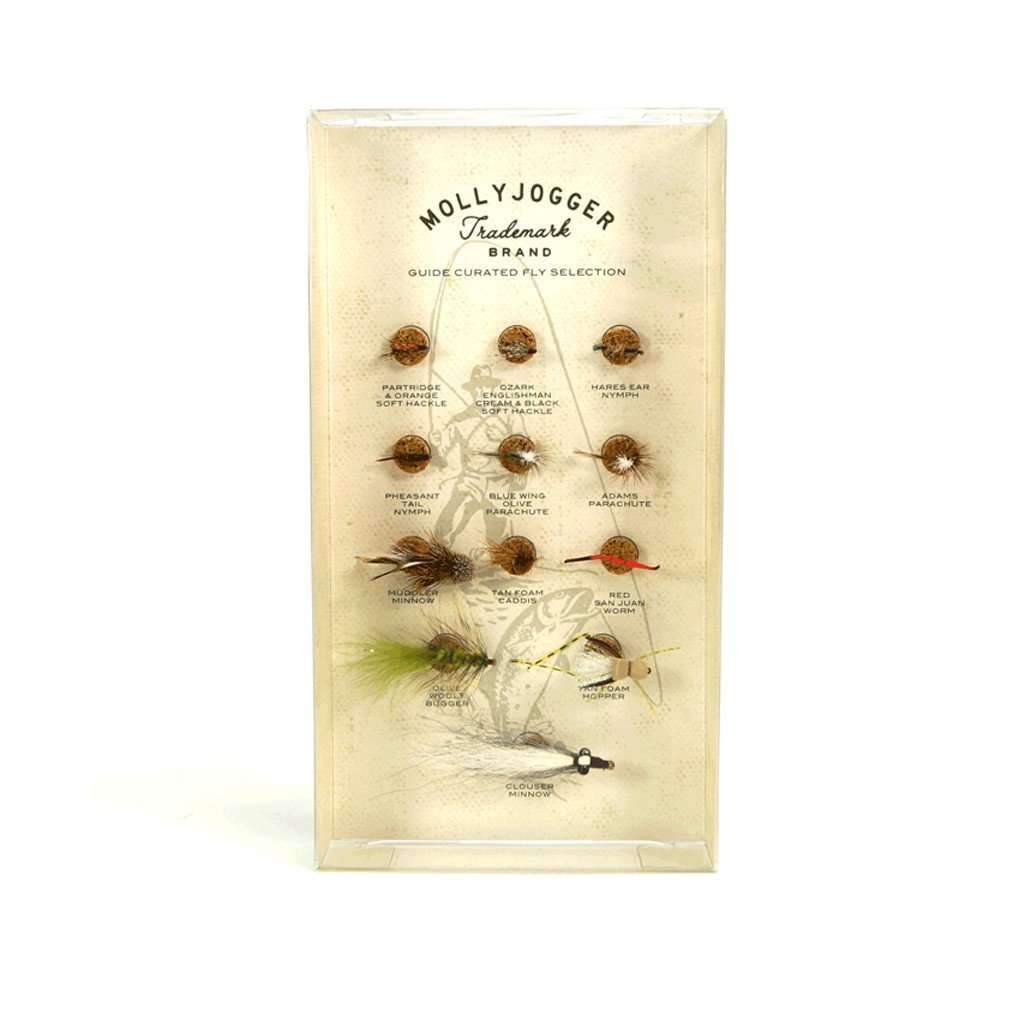This image shows an advertisement for Molly Jogger Trademark Brand Guide Curated Fly Selection. The advertisement is set against a light beige background with a subtle, shadowed watermark illustration of a fly fisherman casting his line. Displayed prominently are 12 intricately designed fishing lures, varying in colors such as white, green, red, and brown. These lures range from simple designs to more elaborate ones crafted with feathers, cork, and other materials. Each lure is meticulously arranged on the placard, which features small, detailed wording describing the brand and the product. The overall appearance suggests high-quality, handcrafted fishing flies intended to effectively mimic insects to attract and catch fish.